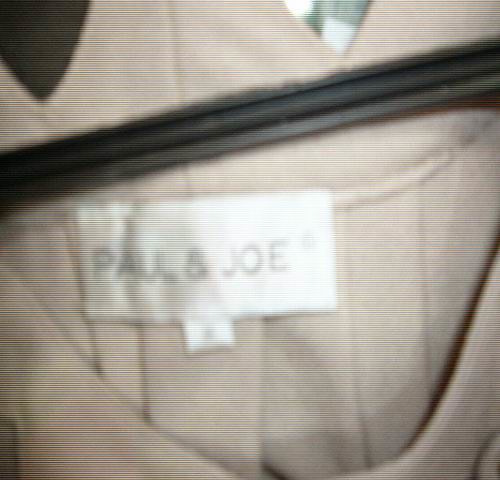This image is a close-up shot of a clothing item, possibly a dress or tank top, that is blurry and difficult to fully discern. The fabric is a light brown to taupe, appearing thin, with various lines running through it that could be pleats or sections. A notable feature is a white tag on the back, which reads "Paul and Joe" in black font. Above the tag, there's a black rectangular element, likely a hanger or part of one, suggesting the clothing is hung up. The neckline appears to be a scoop neck, with unclear sleeve lengths. The garment has a mix of vertical and horizontal lines, adding texture and sectioning to the piece.